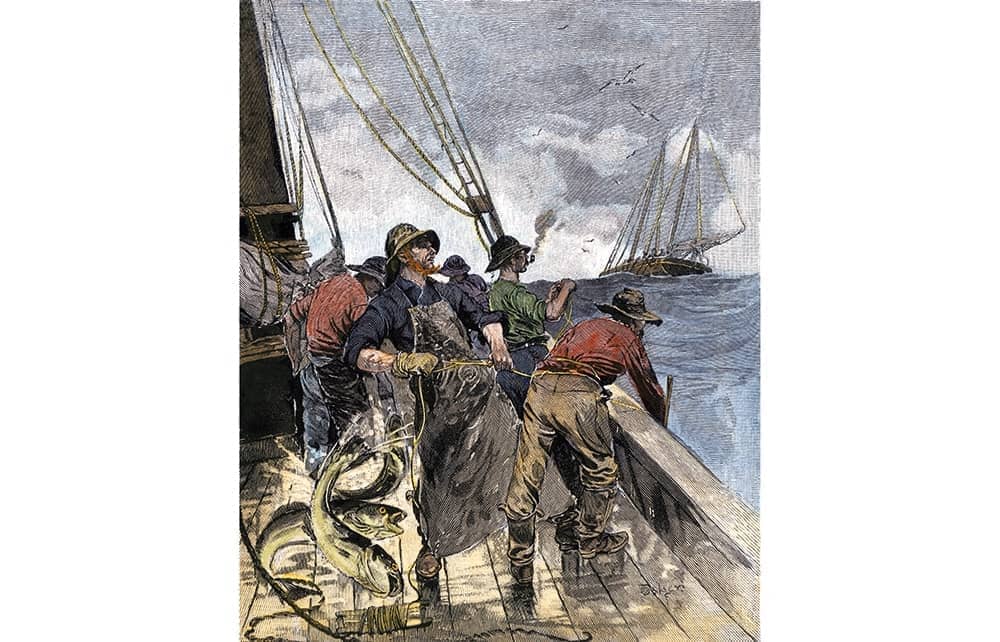The painting depicts an evocative scene of early-day fishing, capturing a moment on a wooden-decked sailboat. At the center, a prominent fisherman wearing a blue shirt, brown boots, a big apron, and a tan poncho hat struggles with a fishing line. Near him, a few white and gray fish are flopping around on the lower left corner of the deck, possibly just caught from the line. Assisting him is another fisherman in a red shirt and tan canvas pants, who is reaching into the water, perhaps to gill the fish. In the background, a fisherman in a green shirt and blue pants stands by the edge of the boat, comfortably smoking a black pipe with gray smoke. Another figure, partly shadowed, wears a black hat, a red shirt, and gray pants. The deck is crisscrossed with tan ropes, enhancing the rustic charm of the scene. The surrounding sea is rendered in varying shades of blue, gray, and white, with high waves. In the distance, a second sailboat, characterized by white sails and a brown hull, traverses the waters. Above, black, gray, and white birds dot the sky, which is similarly hued in white and gray. The painting, signed by the artist in black at the bottom right corner, vividly recalls the bygone era of line fishing under sail, deeply immersing viewers in its nostalgic maritime atmosphere.